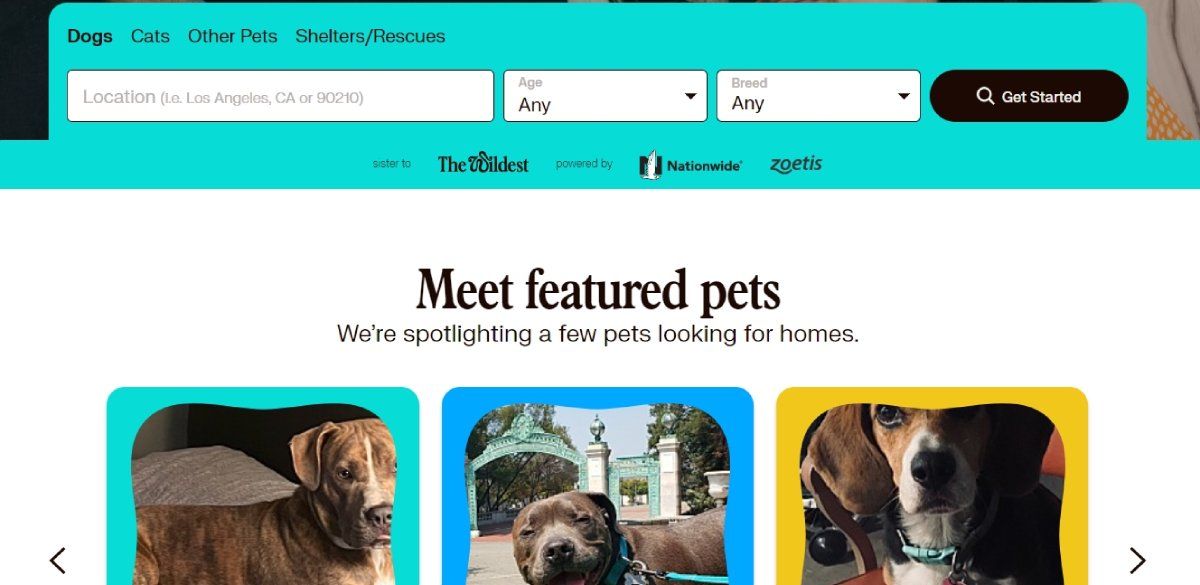This image is a cropped screenshot of the Petfinder website, a platform designed to help users find adoptable pets. The top portion of the page features a large blue navigation bar superimposed on a photo background, with a small cropped preview of the main image visible on the right.

In the top left corner of the blue tab, there are category options for different types of animals: 'Dogs', 'Cats', 'Other Pets', and 'Shelters & Rescues'. The 'Dogs' category is currently selected. Below these options is a large text box labeled 'Location'. In the center of the box within the blue tab, there are two drop-down menus: one for 'Age', set to 'Any', and another for 'Breed', also set to 'Any'. To the far right of these drop-down menus is a prominent black button labeled 'Get Started'. Beneath these options, there are three logos representing the website's sponsors.

The main body of the webpage, which has a white background, contains a centered heading that reads 'Meet Featured Pets'. Underneath is a subheading that says, 'We're spotlighting a few pets looking for homes'. Below the subheading, there are three boxes displaying thumbnails of dogs, highlighting some of the pets currently available for adoption.